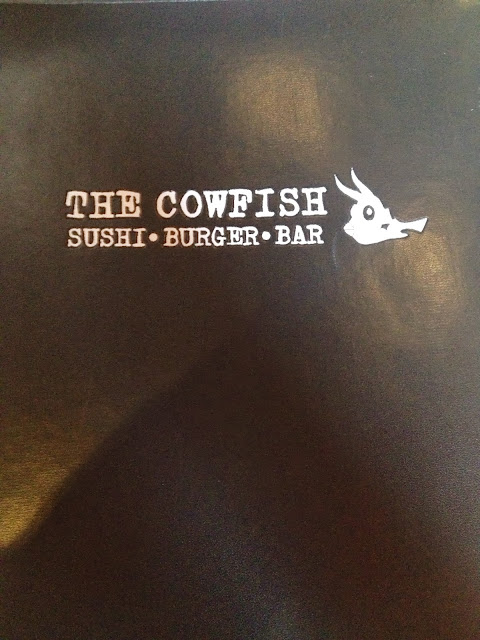The image depicts the cover of a restaurant menu or a sign for 'The Cowfish.' The background is a textured blend of dark browns and tans, giving it a sophisticated, metallic feel, with some light reflections adding depth. Positioned about two-thirds down from the top, the restaurant name 'THE COWFISH' is prominently displayed in large, white, capital letters, resembling an old typewriter font. Below the name, in a slightly smaller white font, are the words 'SUSHI • BURGER • BAR,' separated by dots. On the right side of the text, there is a peculiar drawing of an animal. The sketch appears to be a stylized fish with two horns, facing to the left, featuring prominent black eyes, giving it a unique and artistic touch.